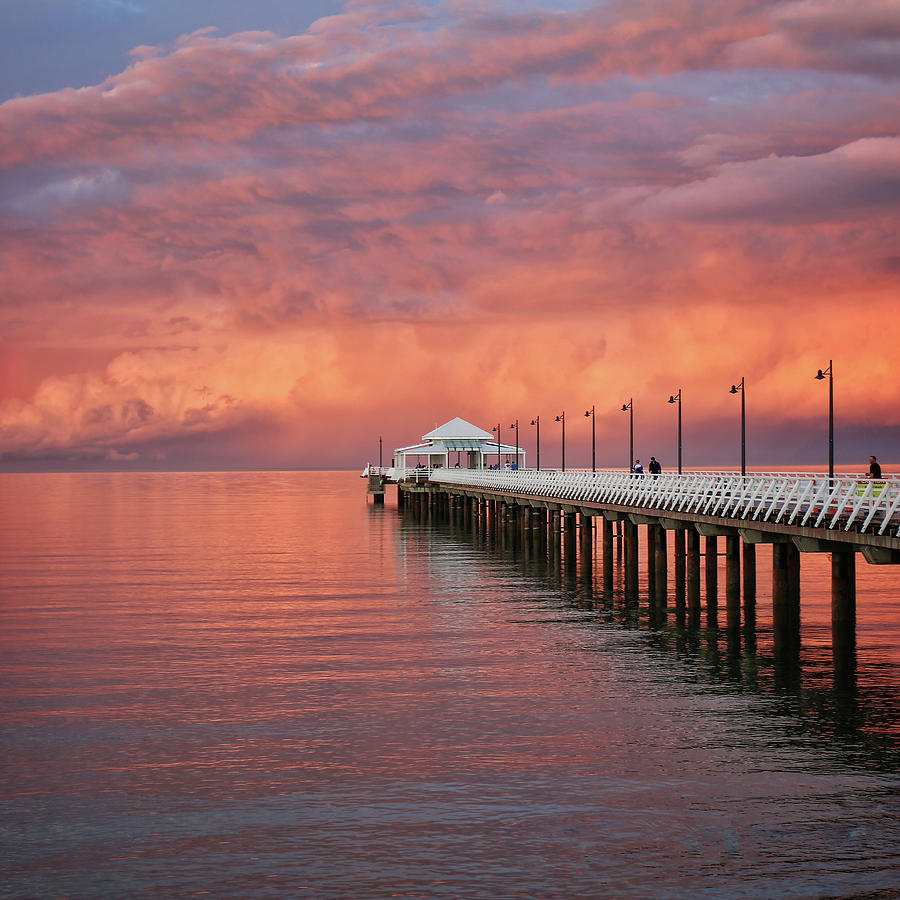The photograph captures a serene outdoor scene during a vibrant twilight, prominently featuring a long pier that extends from the right side into the center of the image. The sky is adorned with incredible shades of pink, purple, and hints of orange and blue, indicative of either a sunset or a heavily polluted day. These vivid colors reflect beautifully on the rippled water, creating a harmonious blend where the water mirrors the sky. The pier is flanked by white guardrails and light poles, which guide the viewer's eye toward a white tent-like structure or gazebo at its far end, situated right at the horizon. A few people can be seen walking along the wooden walkway, adding a human element to this tranquil and picturesque scene.